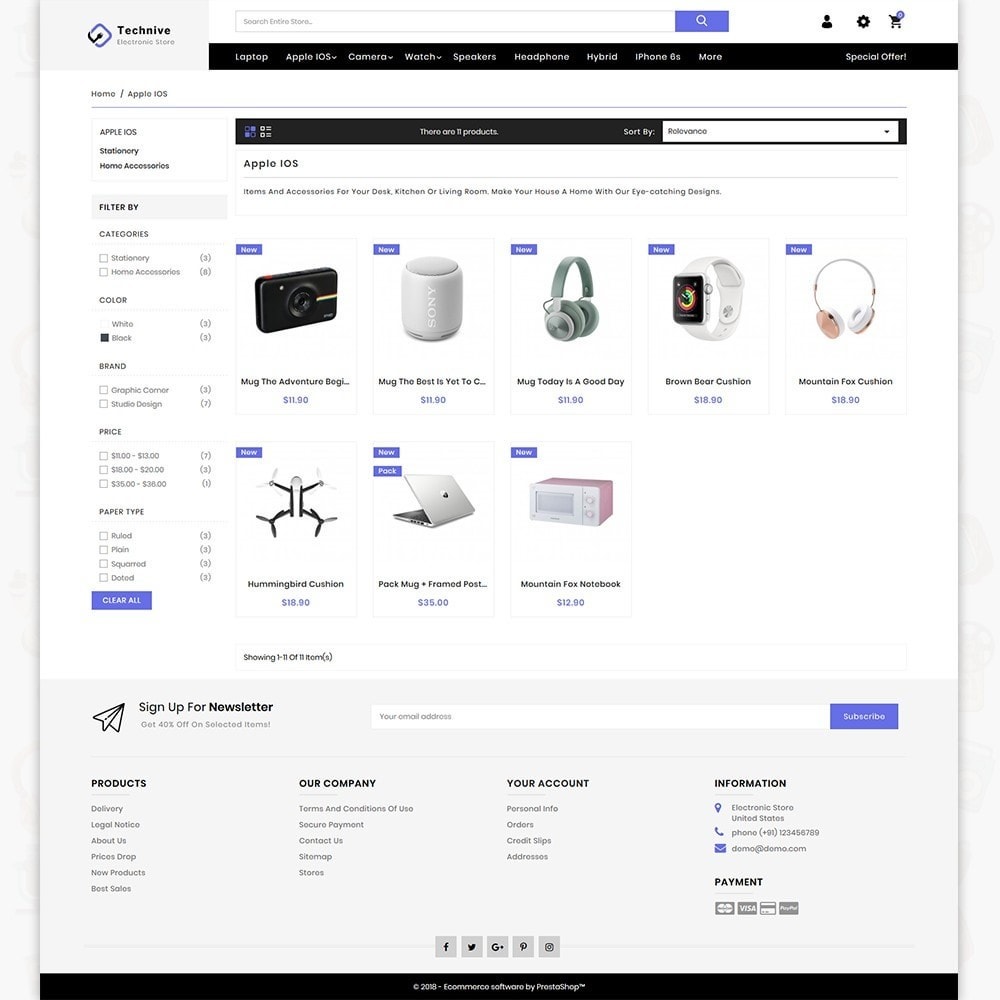This image appears to be a screenshot of a technology-related e-commerce website.

At the very top, the website has a predominantly whitish-gray background with mostly black font and minor white text accents. The header features the title "Top Tech Knives" alongside a blue and black logo that appears to include an electrical cord. 

Directly below, there is a search box accompanied by a purple and white magnifying glass icon. Adjacent to this are three black icons representing a user profile, a settings cogwheel, and a shopping cart, with a small purple notification bubble.

Beneath the header, there is a black navigation bar with submenus categorized into various sections such as "Laptops," "Apple iOS," "Cameras," "Watches," "Headphones," "Hybrid," and more, although some text is blurry and difficult to read. There is also a “Special Offers” section.

Continuing downward, another black bar provides sorting options such as "Search by" and "Relevance," with "Relevance" currently selected. A segment titled "Apple iOS" follows, featuring a brief description.

To the side, there are filtering options where users can refine their search by categories, color, price, etc. This section includes a purple and white "Clear All" button.

The main section displays product images under the "Apple iOS" category, including:
- A retro-looking black camera with a yellow strip,
- A Sony speaker (font is very tiny and blurry),
- Olive-gray headphones,
- A smartwatch with a white band,
- Rose gold and white headphones,
- A black and white drone,
- A silver laptop,
- A pink and white microwave.

Each product image is accompanied by a purple-blue box with white text detailing the items and their prices, although the text is somewhat indistinct.

At the bottom, the webpage provides an option for visitors to subscribe to a newsletter by entering their email address. Additional submenus include "Products," "Discovery," "Legal Notice," "About Us," "Blog," and others. Details about "Our Company" such as "Your Account" options, contact information (address, phone number, email), accepted payment methods (MasterCard, Visa, etc.), and social media icons (Facebook, Twitter, etc.) are listed. The page concludes with copyright information.